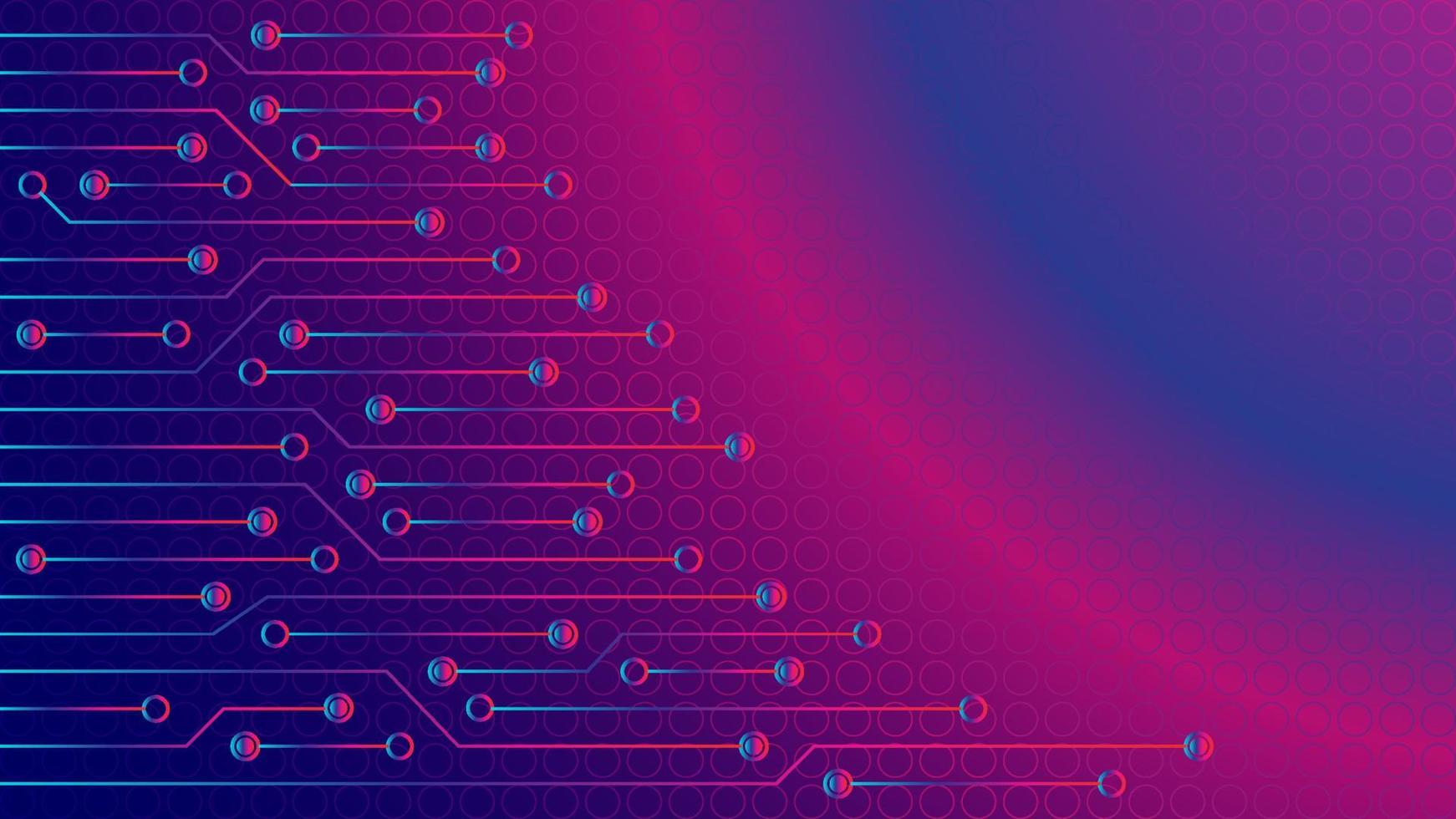The image is an abstract, digitally created design, possibly a desktop wallpaper, dominated by shades of blue, purple, pink, magenta, and fuchsia. The background starts as a deep blue on the top right corner, forming a triangular shape that transitions to a misty, light red, and then back to blue, extending to the left edge. On the left side, various rods with small circular nodes are present. Some rods are straight, while others zigzag, featuring either open or filled circles. These rods and nodes vary in color but maintain a consistent palette of blues, purples, and pinks. The composition includes additional lines, some resembling quarter circles, stretching from left to right as they descend in the image, contributing to the complex, vibrant pattern. The design overall is highly abstract, lacking any text or discernible objects, and showcases a sophisticated interplay of colors and shapes.